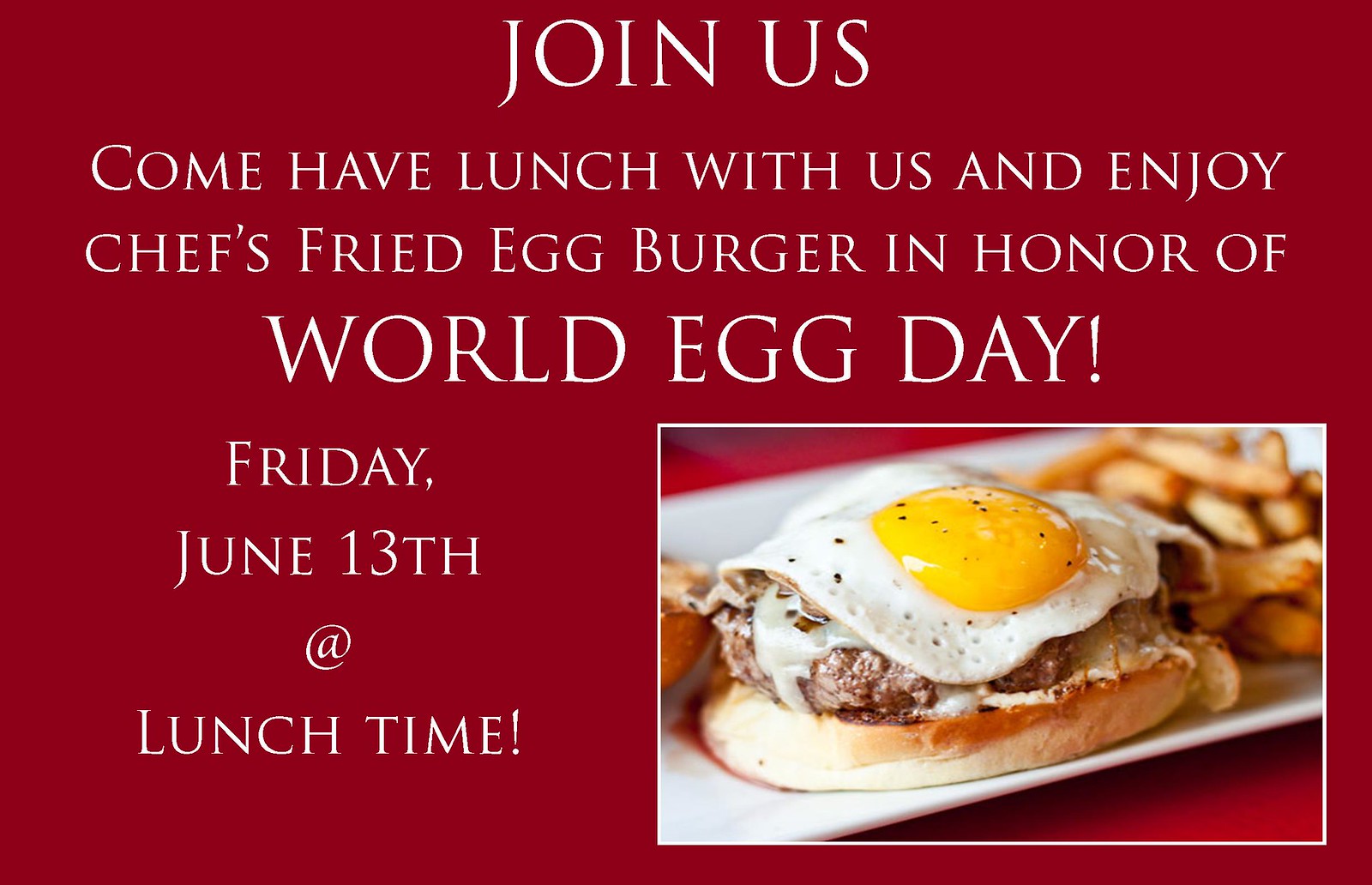The image displays a horizontally oriented flyer with a deep, dark red background, advertising an event for World Egg Day. In prominent white letters, it invites viewers to "Join Us," encouraging them to "come have lunch with us and enjoy Chef's Fried Egg Burger in honor of World Egg Day, Friday, June 13th at lunchtime." 

On the lower right-hand corner of the flyer, there is a detailed photograph of the featured dish. The dish is presented on a white plate, which begins to blur towards the back. The photo highlights a hamburger bun supporting a beef patty layered with caramelized onions and white cheddar cheese, all crowned with a sunny side up fried egg generously sprinkled with black pepper. Next to the burger, a pile of French fries is visible, although out of focus, directing the viewer's attention to the appetizing egg with its runny yolk.